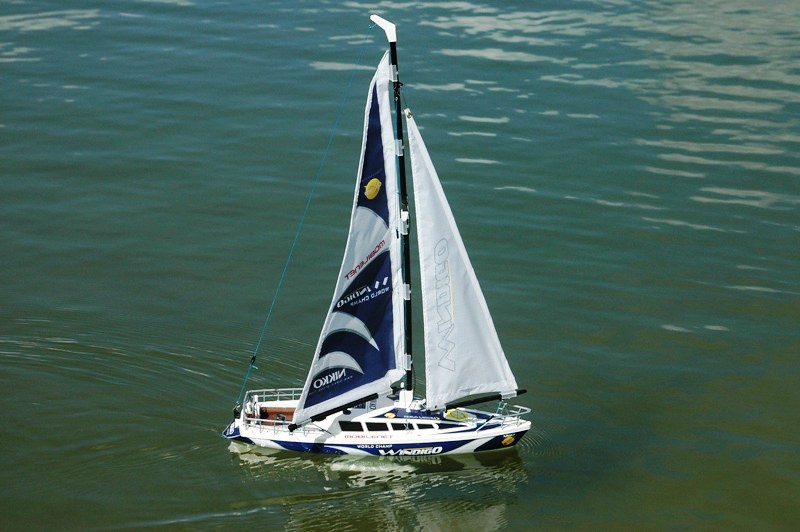This is a full-color, daytime photograph taken outdoors, featuring a calm body of water with a few gentle ripples. The water has a greenish-brownish hue, suggesting it's not the cleanest, and it is most likely a lake. The focus of the image is a toy remote-operated sailboat, which is evident from the way the ripples move around it. The boat is primarily white with navy-blue accents. It has two sails: one all white and the other blue and white. The sailboat is positioned facing rightward. Prominently displayed on its side in white text is the name "Windigo," which is slightly misinterpreted in different accounts but consistently identified. There is some additional text on the sails that is not fully legible, but parts of it seem to spell out "NIKKO." The overall serene scene includes a partial reflection of the sailboat in the greenish water, enhancing the tranquil ambiance.